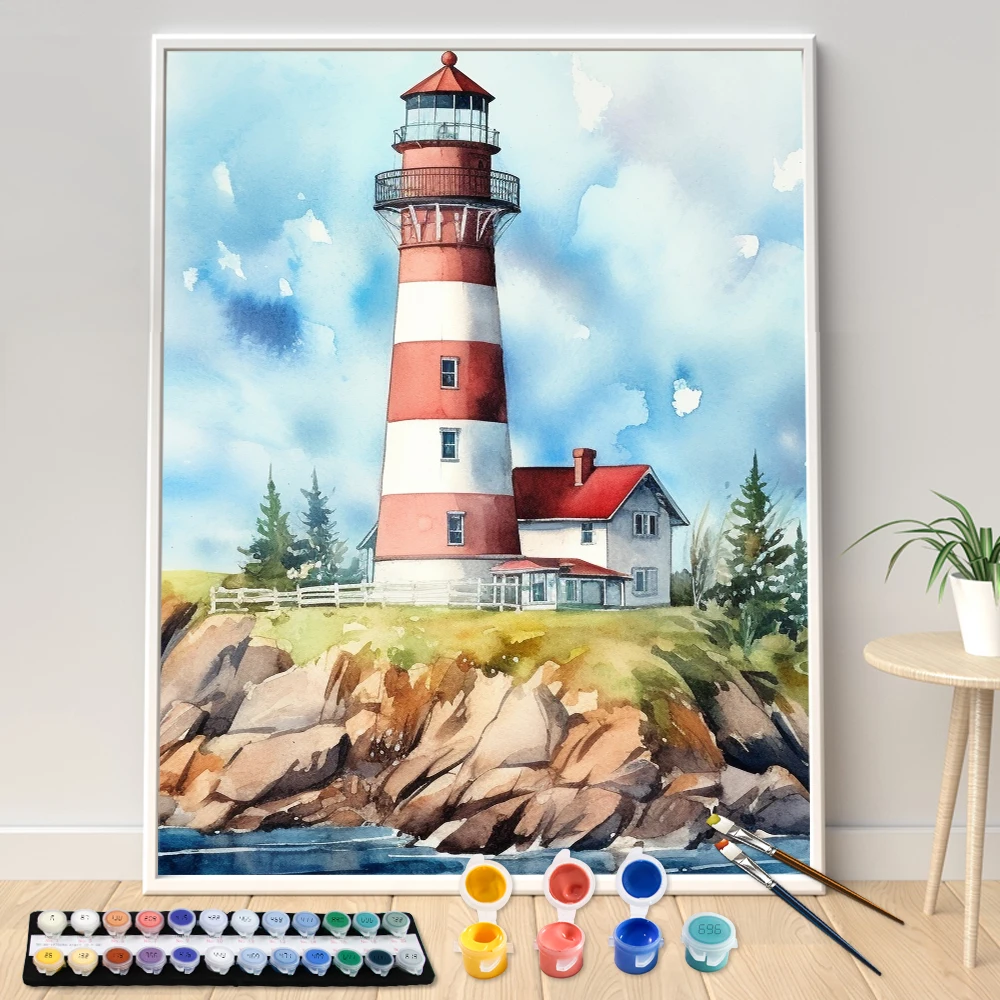This detailed image captures a nearly completed paint-by-number artwork of a picturesque lighthouse scene. The lighthouse, adorned with thick red and white stripes, stands on a rocky seaside hill. Its red-domed top features glass encasing and a black wrought iron catwalk. Adjacent to the lighthouse is a quaint white house with a red roof, surrounded by pine trees and a fenced yard. The rocky terrain descends to the blue sea, set against a mottled sky in various shades of light to dark blue. 

In the foreground, the painting is displayed on a table, with an open paint kit to the left including a specific tray of colors used for the house. There are three open pots of paint—yellow, red, and blue—alongside two paintbrushes, each tipped with paint. To the right of the scene, there's a three-legged accent table with a white pot holding a green spider plant. This comprehensive setup illustrates the artistic process in action, blending real elements with the vibrant visual of the paint-by-number lighthouse.